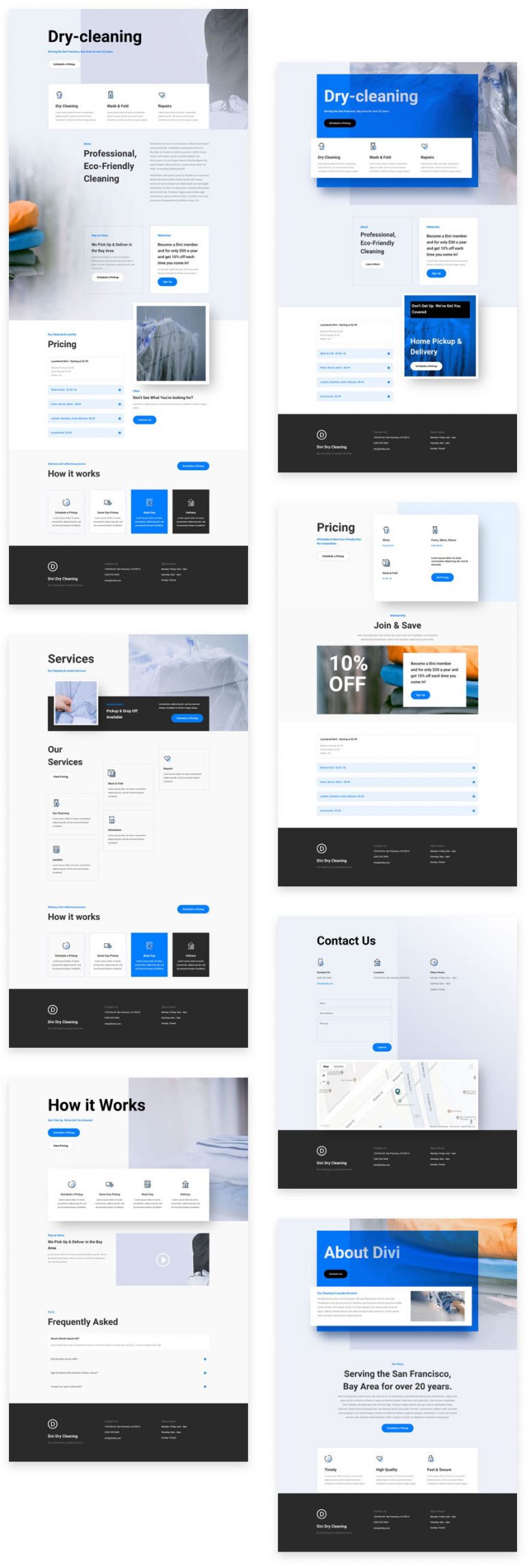This image features a detailed, segmented layout presenting information about a dry cleaning service. The layout is divided into seven distinct sections:

1. **Dry Cleaning Services**: The first section introduces the dry cleaning services available, featuring a blue box with some personal information redacted for privacy. 

2. **Services Overview**: Positioned on the right, it details various dry cleaning services. This section includes an icon of a dry cleaning bag draped over a garment and a pricing menu.

3. **Pricing and Discounts**: This part offers a pricing menu which prominently displays a 10% discount offer. The discount is placed atop a vibrant graphic with orange and blue hues that make it eye-catching.

4. **Contact Information**: Below the pricing section, this area provides multiple contact methods for clients to get in touch with the service providers.

5. **How It Works**: Moving back to the left, there's a section explaining the step-by-step process of how the dry cleaning service operates, ensuring clarity for potential customers.

6. **About Us**: On the right-hand side, an "About" section is highlighted in blue, sharing detailed information about the company or service providers.

Each section is methodically designed to provide comprehensive information, ensuring potential customers have all the necessary details about the dry cleaning services, including how they work, their offerings, and how to get in touch.